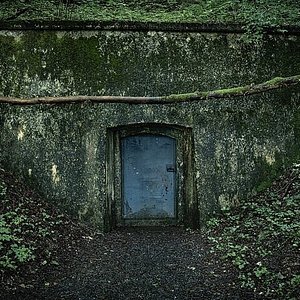The image is a perfectly square photograph, most likely of an old concrete wall now covered extensively in mold and green moss. At the top of the wall, a patch of greenery, possibly grass or more moss, is visible. Traversing the image horizontally just above the center is what appears to be either a tree branch or a rope. In the very center of the image is a recessed doorway featuring a dark blue door. Emerging from this door is a pathway composed of dark mulch or dirt that extends downward toward the bottom of the image. Surrounding the pathway, on both the left and right sides, are various green shrubs and foliage, contributing to the overall overgrown and abandoned atmosphere of the scene. Green and white streaks on the wall add to its textured and aged appearance. The only significant color comes from the dark blue door, while the rest of the image is dominated by dark hues of black and green, giving it a somewhat mysterious and eerie feel. No text or people are present in the image, heightening its enigmatic and solitary ambiance.